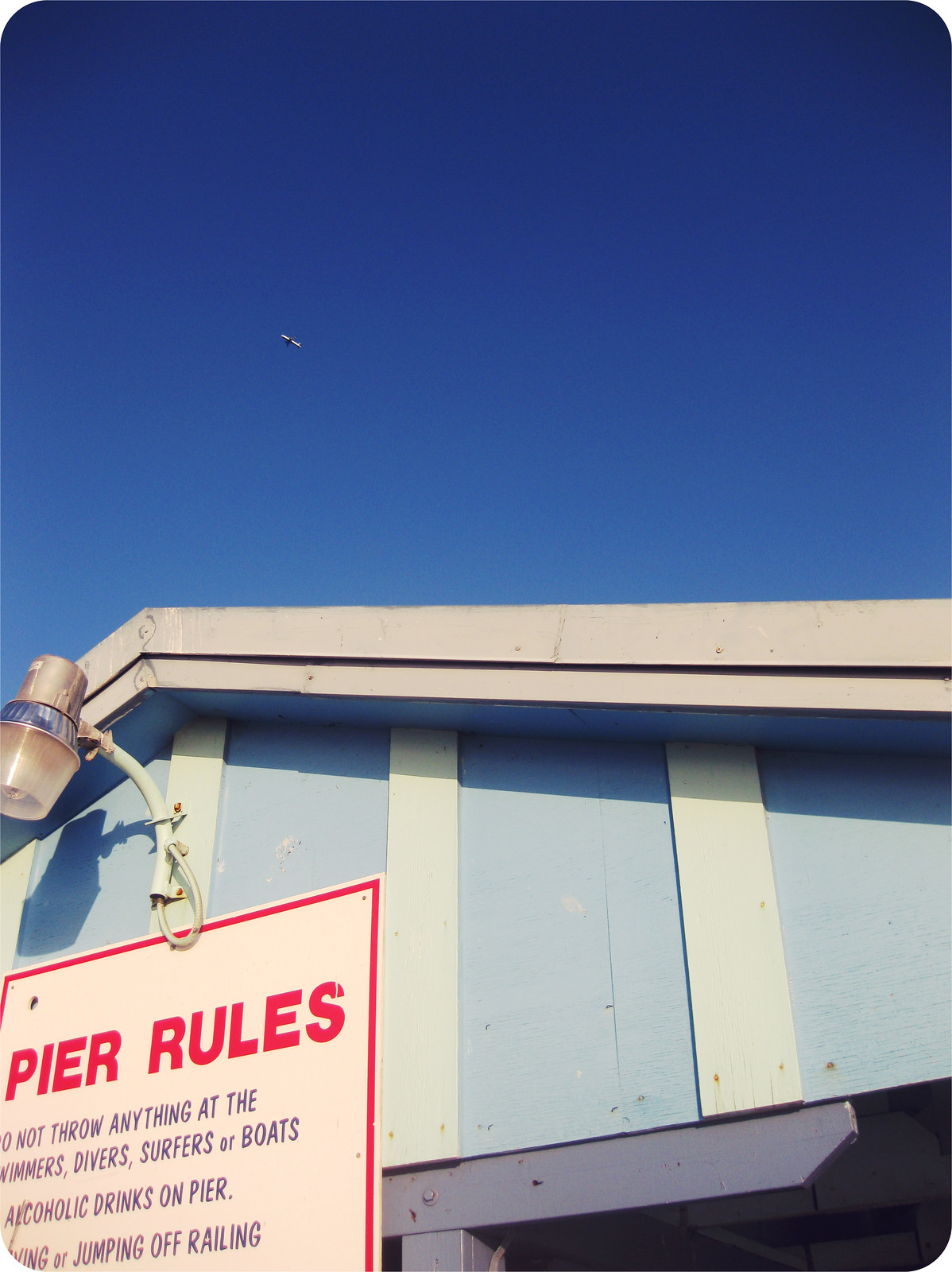This captivating photograph showcases the triangular roof of a pier against a backdrop of a crystal clear, nearly navy blue sky, with a small airplane ascending in the distance. The foreground is dominated by the right side of the building’s V-shaped roof, adorned with a curved light fixture that's not turned on. Below the light, a white sign with a red border prominently displays the "Pier Rules," including regulations against littering, drinking alcoholic beverages, and throwing objects at swimmers, divers, surfers, or boats. The building itself features blue with white vertical panels, adding a striking contrast to the scene. The image, devoid of clouds, emphasizes the pier's serene yet structured environment.